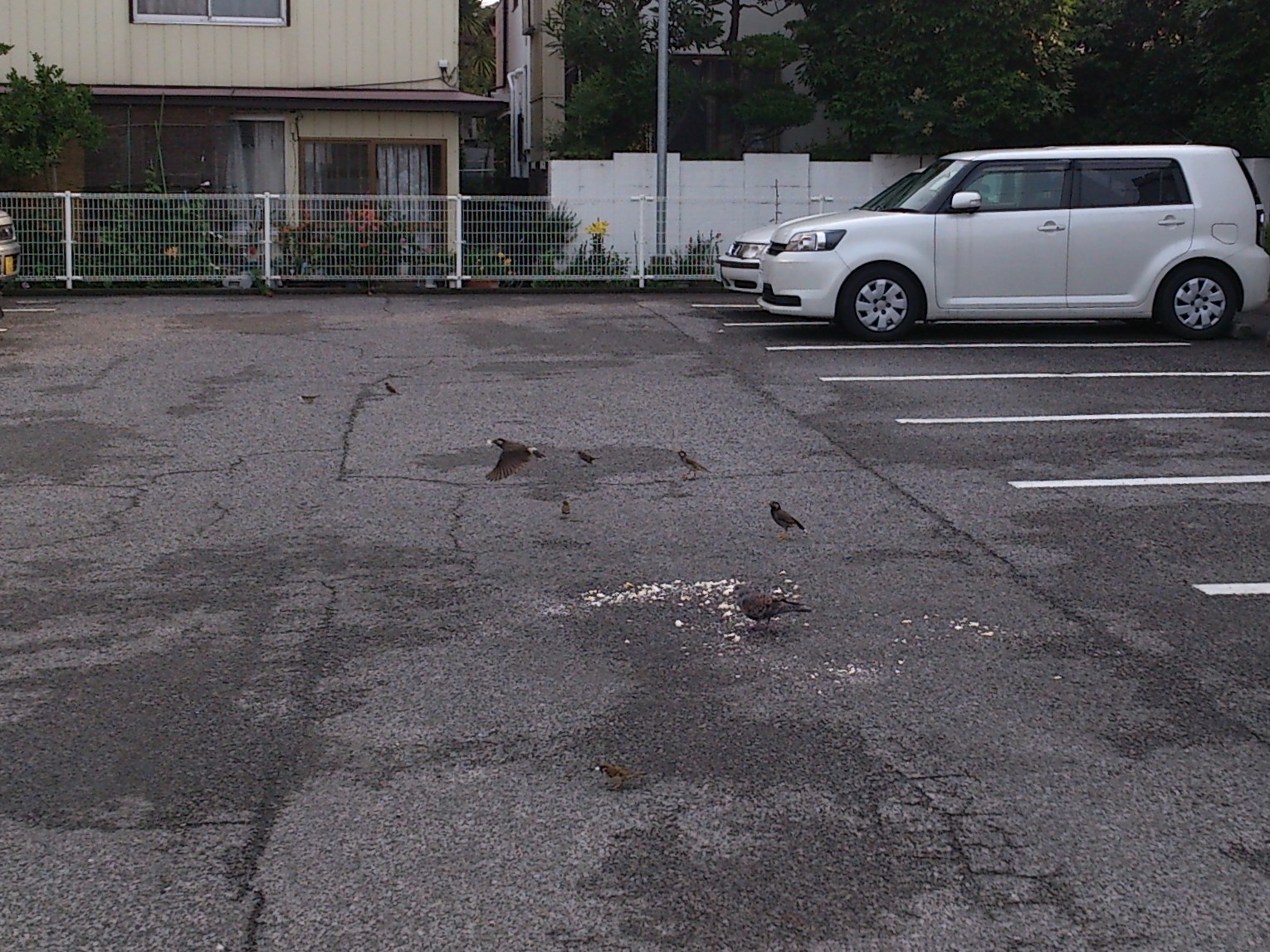This outdoor scene captures a somewhat neglected parking lot with several notable features. The lot, which is badly in need of repaving, has several visible cracks and oil patches. There are defined white parking spaces along the right side, occupied by a white SUV and a white sedan. In the distance, a silver hatchback is also parked. At the center of the image, a group of brownish-black birds are scavenging crumbs, possibly bread, scattered on the pavement. Surrounding the parking lot, a metal fence encloses the area, and to the right, there is an alleyway leading to other buildings.

In the top half of the photo, two residential buildings are partially visible. The house on the left has a yellowish-tan hue, with a window on the top left and a door with bars on the ground level. This house is fronted by a garden containing various green plants and flowers, including yellow and pink blossoms. Trees with lush green foliage obscure parts of the buildings and extend to the right of the scene. Despite the overall overcast lighting, the greenery stands out in vibrant contrast to the grey, worn parking lot below.